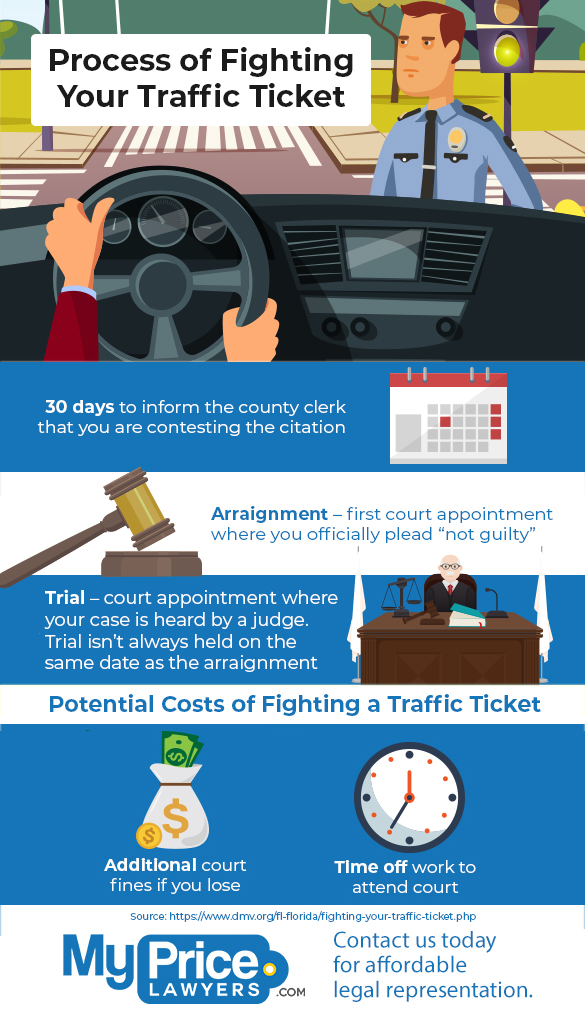The infographic titled "Process of Fighting Your Traffic Ticket" features a detailed, cartoon-style illustration and step-by-step guide on how to contest a traffic ticket. At the top, a white rectangle with black text displays the title. Below it, a 3D cartoon graphic showcases the interior of a car with a Caucasian driver holding the steering wheel, and a Caucasian police officer standing near a traffic light at an intersection. The visual elements are framed by a blue horizontal bar highlighting key steps in bold white text: "30 days to inform the county clerk that you are contesting the citation," accompanied by a calendar with circled dates.

Further down, another section explains the legal process: "Arraignment - first court appearance where you officially plead 'not guilty'," illustrated by a gavel striking a block. This is followed by, "Trial - court appointment where your case is heard by a judge. Trial isn't always held on the same date as the arraignment," supplemented by a cartoon drawing of a judge at his bench, complete with scales of justice, a wooden desk, and a gavel. The judge is depicted wearing a black robe, with gray hair and glasses.

The infographic then outlines the potential costs involved in fighting a traffic ticket. It lists "additional court fines if you lose," represented by a money bag with bills sticking out and a gold dollar symbol, and "time off work to attend court," symbolized by a clock with red hands. The bottom section, framed by white and blue bars, reads "MyPriceLawyers.com" with "Contact us today for affordable legal representation."

This infographic effectively combines text and visuals to guide the viewer through the process of contesting a traffic ticket while highlighting essential time frames, legal steps, and possible costs.